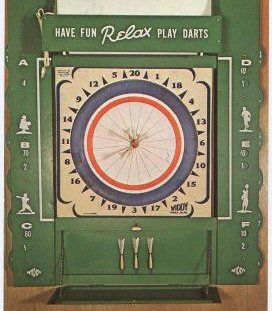This vintage dartboard, likely from the 1940s or 50s, is framed in a hunter green wooden case. The board's target area features concentric rings: a white innermost circle, circled by an orange band, followed by a blue band. Around the blue band are different scoring sections, akin to a clock, marked with numbers like 20, 18, 13, and 4. The dartboard shows signs of extensive use over the years. Flanking the dartboard on either side are white silhouettes of sports players, including figures playing baseball and basketball, among others. Positioned above the dartboard is a sign that cheerfully encourages, "Have fun, relax, play darts." Additionally, three white darts are mounted on the board. The entire set is housed within what appears to be an old-fashioned wooden cabinet, likely on a light brown background.